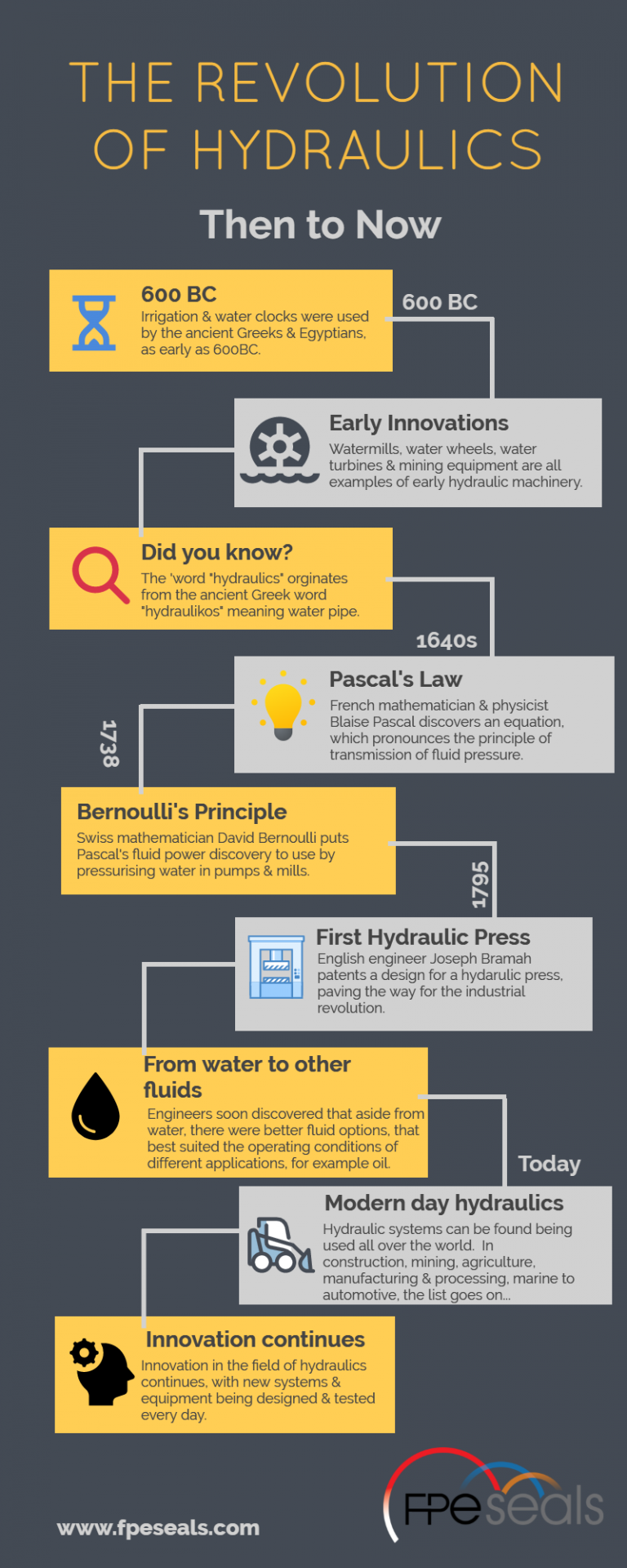This visually striking, vertical-print piece serves as an informative flow chart on the evolution of hydraulics, stretching from 600 BC to the modern day. It features a dark gray background without a border and is considerably taller than it is wide. The topmost part of the image features the title "The Revolution of Hydraulics" in bold gold text, followed by "Then to Now" in gray text. The flow chart is composed of horizontally rectangular boxes that alternate in color between gold and gray, each containing a symbol, a date, or a description. 

The progression begins with an hourglass symbol accompanied by "600 BC," highlighting early innovations like irrigation and water clocks used by ancient Greeks and Egyptians. The next gray box reads "Early Innovations," showcasing examples like water mills, water wheels, and mining equipment. The subsequent gold box, stating "Did You Know?" explains that the term "hydraulic" originates from the ancient Greek word "hydrolysis."

Following this introductory phase, the flow chart moves through significant milestones: the 1640s with "Pascal’s Law" discovered by French mathematician and physicist Blaise Pascal, and 1738's "Bernoulli’s Principle," identified by Swiss mathematician Daniel Bernoulli. The year 1795 marks the invention of the first hydraulic press, as denoted in another gold box.

The timeline continues with advancements "From Water to Other Fluids," leading to today’s "Modern Day Hydraulics," which is a gray box labeled "Today." The piece concludes with an optimistic note in the final gold box, stating "Innovation Continues." This comprehensive visual narrative encapsulates the rich history and ongoing development of hydraulic technology.